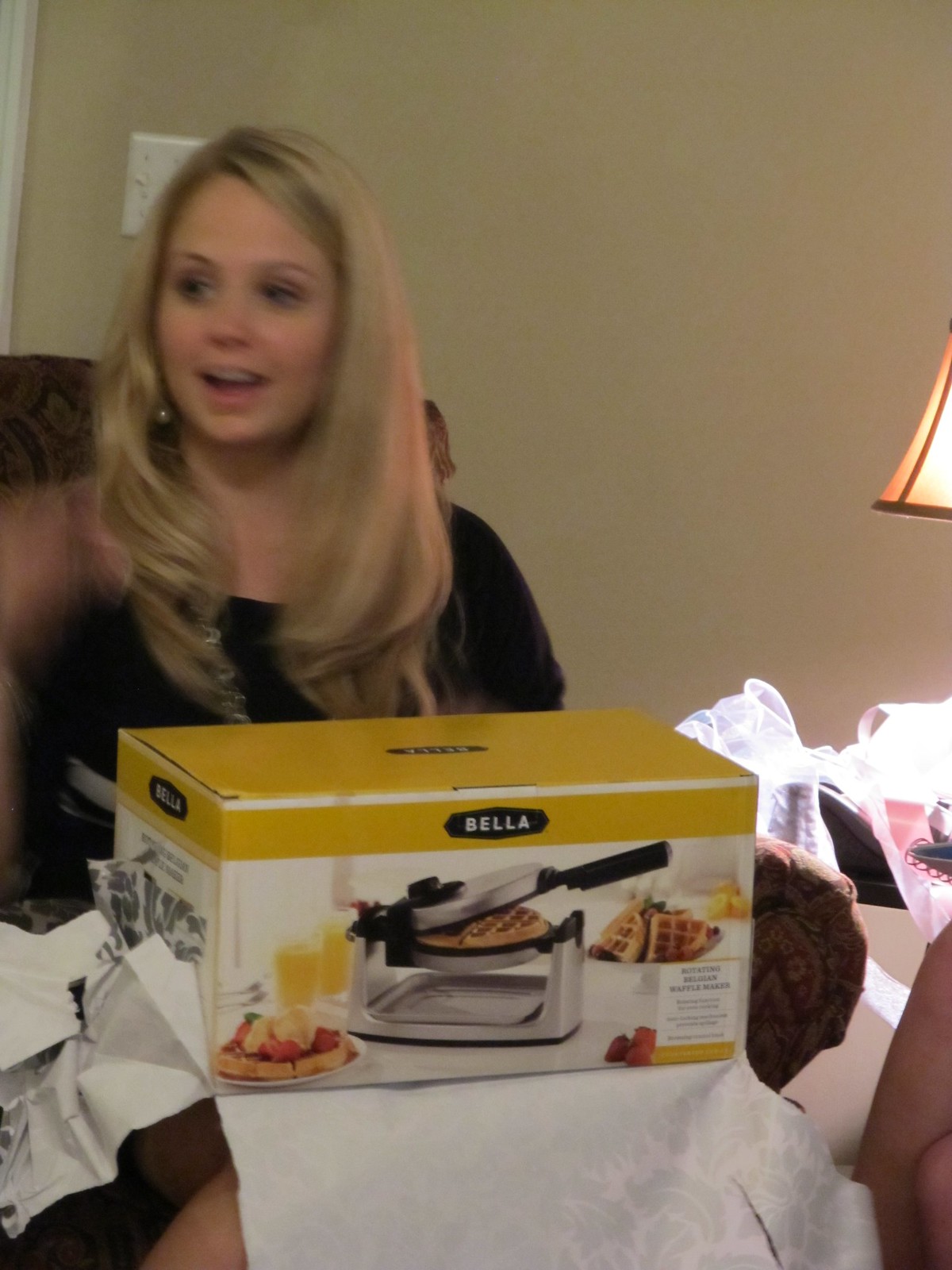In this image, a young blonde woman in her mid-twenties, wearing a stylish black shirt with sheer sleeves, is opening a gift that appears to be a Bella brand waffle iron. The unopened yellow box, which has wrapping paper draped around it, rests on her lap. The box features the Bella logo, an image of a waffle iron with a waffle inside, and various serving suggestions including strawberries, fruit, and butter. The scene suggests a celebratory event, possibly a wedding shower, as the woman is well-groomed and there are decorative bows around, indicating it’s a special occasion. She is seated on a dark-patterned chair, and a lampshade is partially visible to the right, casting a warm light. The background displays a dark beige wall and a white light switch panel, partially obscured by her head, adding to the cozy domestic setting. Nearby, the legs of another person can be seen crossed on a different chair, suggesting she is not alone.